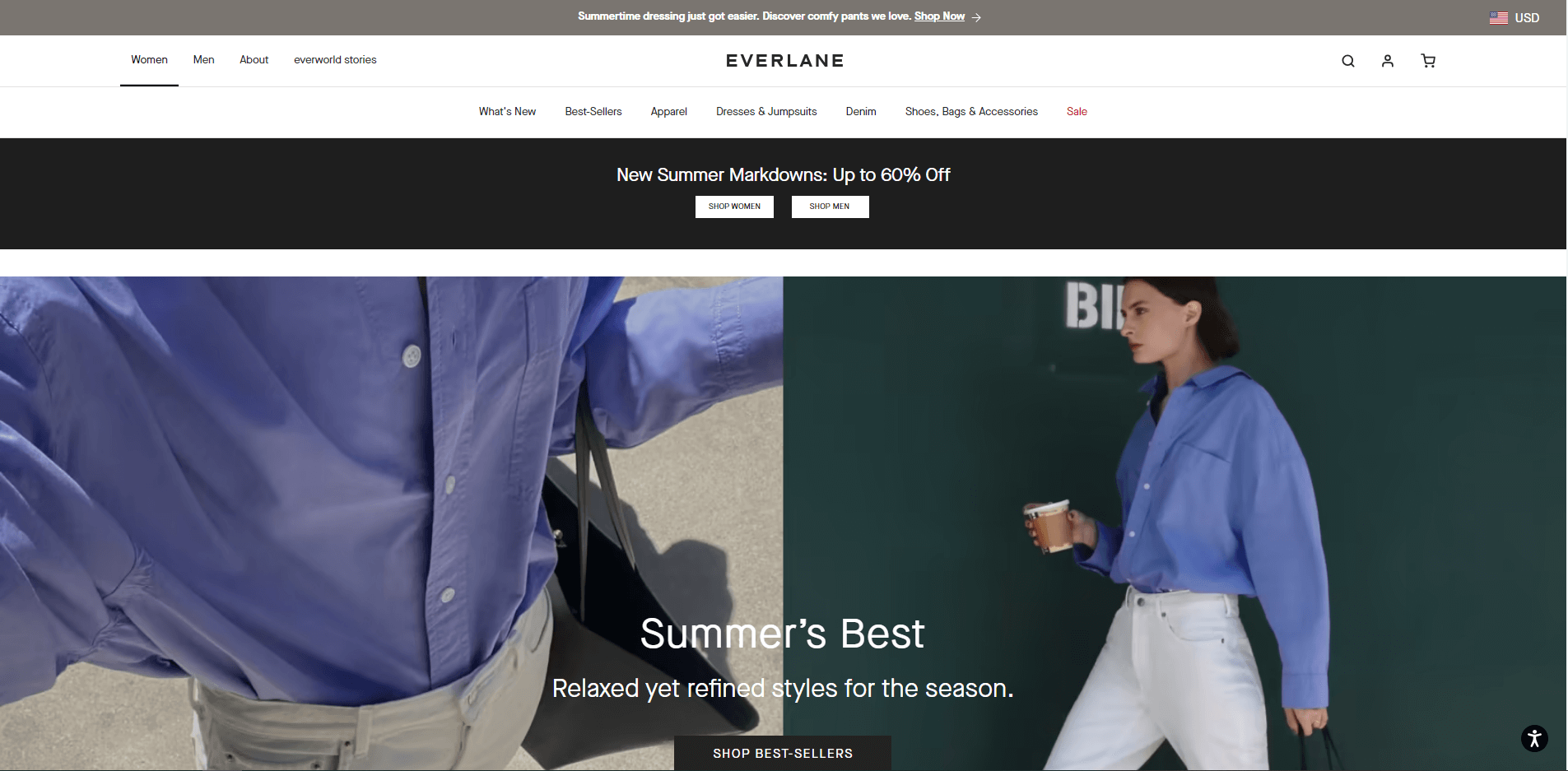The image is a screenshot from the Everlane website. At the top center, the Everlane logo is prominently displayed. To the left of the logo, there are navigation links labeled "Women," "Men," "About," and "Everworld Stories." To the right, there are icons for search, user profile, and shopping cart functionalities.

Underneath these navigation options, the next line features additional categories like "What's New," a blurry label, "Apparel," and others, concluding with "Shoes," "Bags," and "Accessories." A red-text button indicating a sale is also visible in this section.

The subsequent section is marked by a large black rectangle with the text "New Summer Markdowns Up to 60% Off." Below this, there are two interactive buttons.

The following section showcases two images of the same person. On the right-hand side, the individual is captured walking, while the left image displays them posing to highlight their outfit. Accompanying these photos is the text: "Summer's Best Relaxed Yet Refined Styles for the Season."